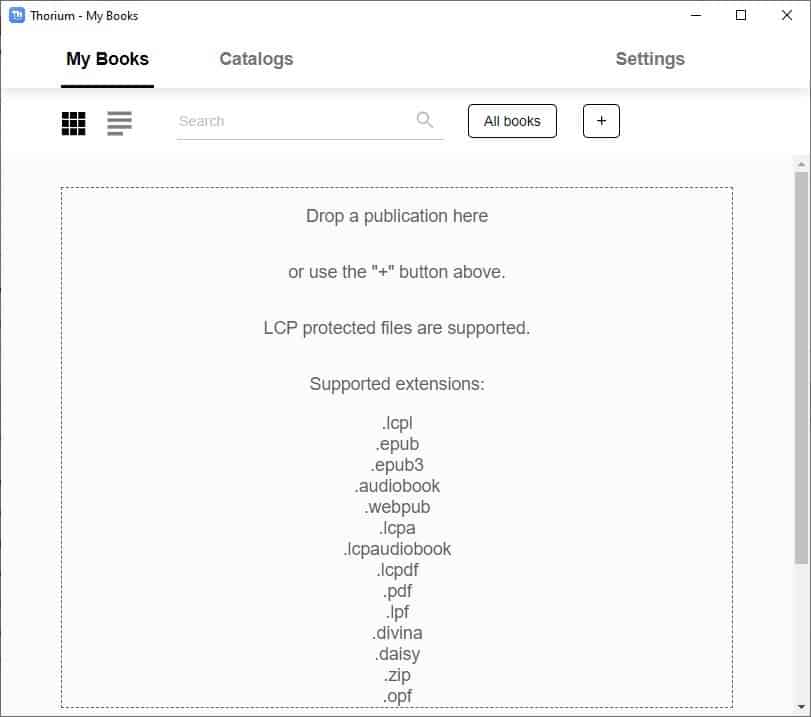Top left corner of the interface displays the words "Thorium, My Books," alongside a blue square containing white shapes. On the top right, you can see the standard window control icons: "X," "square," and "dash." Below the top-left label "My Books" in bold black text, there are three additional labels: "Catalogs" to the right of "My Books," a blank space, and then "Settings" on the far right.

In the middle section, there's a search bar, and to its right, enclosed in a box, is the label "All Books" with a smaller box containing a plus symbol next to it. Below the search bar, inside a larger boxed area, several lines of text are vertically arranged. These lines read: "Drop a publication here," "or use the plus button above," "LCP protected files are supported," followed by "Supported extensions." The supported file extensions listed are: LCPL, EPUB, EPUB3, Audiobook, WebPub, LCPA, LCPA Audiobook, LCPDF, PDF, LPF, Divina, Daisy, Zip, and OPF.